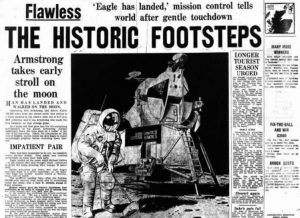The image depicts a black-and-white newspaper front page from 1969, capturing the historic moment of Neil Armstrong's first steps on the moon. Prominently displayed at the top of the page, the headline reads, "Flawless: An Eagle Has Landed," followed by the subheading, "Mission Control tells world after gentle touchdown." A central photograph shows Neil Armstrong standing next to the lunar module on the moon's surface. The headline further announces, "The Historic Footsteps: Armstrong Takes Early Stroll on the Moon." Additional columns of text flank the image, with one visible headline reading, "Longest Tourist Season Urged." The bold, deep black fonts make the headline and key phrases stand out against the white background, accentuating this monumental achievement in space exploration.